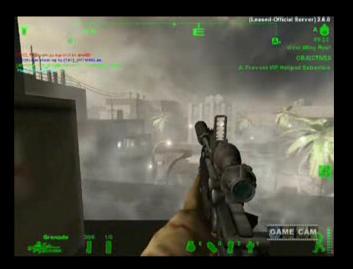The image is an in-game screenshot from a video game, featuring the player's viewpoint in a battle-torn urban setting. The player character, centered in the image, is holding a sniper rifle with a visible sight, his gloved left hand gripping the weapon. The environment is filled with wispy, smoky clouds, suggesting camouflage or places to hide. Buildings and factories are seen on the left, and there appears to be a wall in the lower left corner. The right side features what might be palm trees and more buildings shrouded in smoke. Several green icons indicating weapon types and ammunition are lined up at the bottom of the screen. Additional green text providing detailed analysis is present in the top right corner, with a potential chat window in the top left for notifications. The bottom right corner contains a small caption that reads "game cam," emphasizing the immersive shooter viewpoint. The entire image is bordered by a wide black frame, enhancing its rectangular shape. The central building appears to be gray and has roughly three levels, but no other characters are visible in the scene.